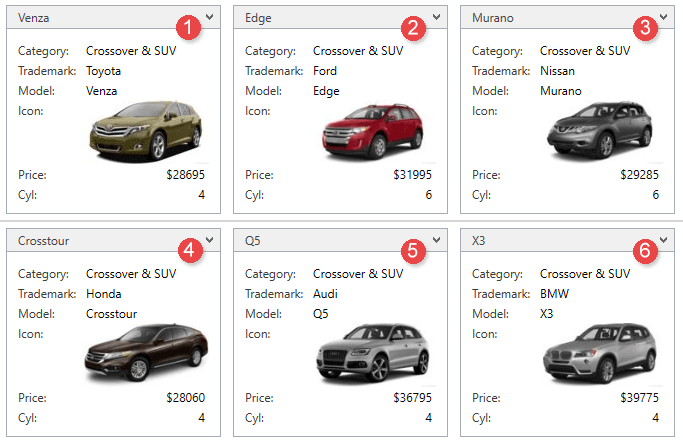The image depicts a horizontally rectangular frame showcasing a grid of six cars arranged in two rows of three. Each car's image is housed within a square. The squares are numbered sequentially with red circles situated in the upper right corners, labeled from 1 to 6 in a left-to-right, top-to-bottom order.

The vehicles displayed are as follows:
1. **Venza** ($28,695)
2. **Edge** ($31,995)
3. **Murano** ($29,285)
4. **Crosstour** ($28,060)
5. **Q5** ($36,795)
6. **X3** ($39,775)

Each square provides detailed information about the respective vehicle, including the category, trademark, model, an icon representation, and an image. The number of cylinders for each vehicle is also mentioned, aligning with the price details for an informative product item page experience.